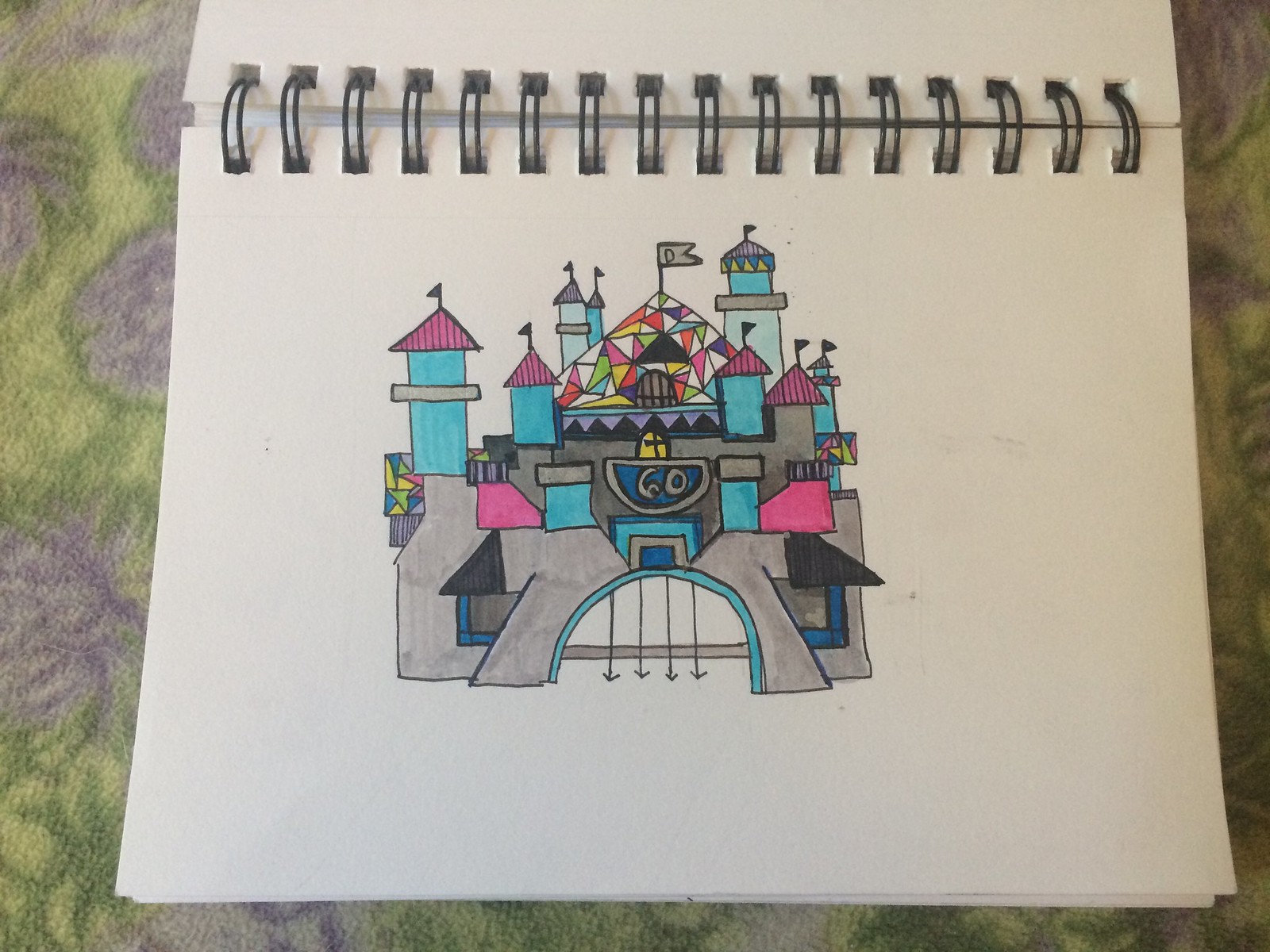This illustration, created with colored pencils or crayons, depicts an ancient castle adorned in vibrant pastel hues. The central structure features tall pillars and overlooks, intricately detailed in various shades. At the forefront and near the base of the building, there is a prominent semi-circular gateway, highlighted by four gray or black arrows pointing downward, possibly indicating the entrance or its gate bars. Situated above this gateway is a semi-circular section with a blue background, encased within a gray border, showcasing the number "6060" in gray text. Further up, a black Christian cross stands prominently. Crowning the castle is a mosaic-patterned triangle or pyramid, beautifully composed of white, green, yellow, and pink pieces. The overall scene blends historical architecture with a lively palette, creating a captivating visual narrative.